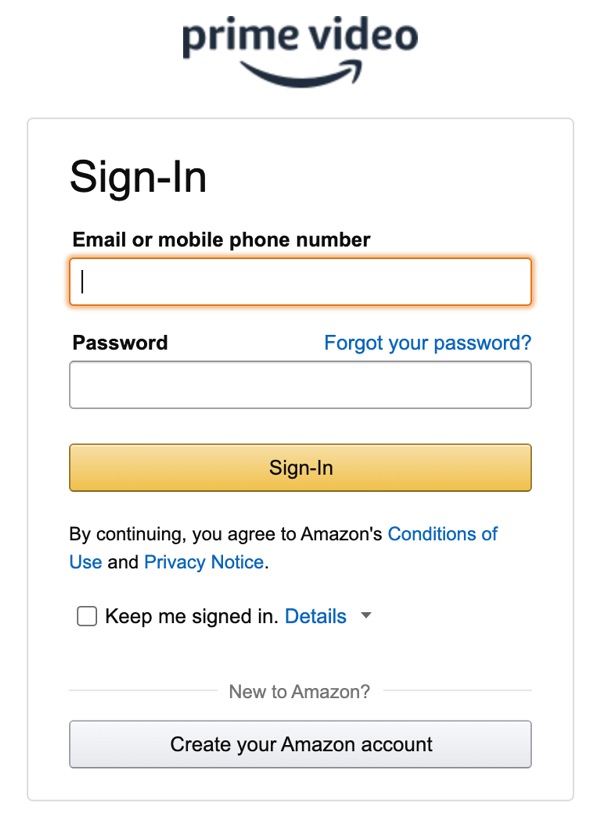The image is a screenshot with a predominantly white background, seemingly captured from a mobile app interface, most likely Prime Video. At the top of the screenshot, the Prime Video logo is displayed in lowercase letters, accompanied by the familiar smirking smiley face logo.

Beneath the logo, a gray-bordered rectangular box contains the login interface. At the top of this box, the bold text "Sign In" is displayed. Just below this, in smaller text, it prompts users to input their "Email or Mobile Phone Number." An input field with a yellow border, presently active with a blinking cursor, is provided for this purpose.

Following the email input field, the phrase "Forgot Your Password?" is shown in blue text, serving as a clickable link. Below this, there is another input field designated for the password entry. Toward the bottom of this section, a gold-yellow button displayed prominently reads "Sign In."

Below the sign-in button, a disclaimer informs users that "By continuing, you agree to Amazon's Conditions of Use and Privacy Notice." Additionally, there is an option to remain signed in by ticking a checkbox labeled "Keep me signed in."

At the very bottom of the gray-bordered box, another section labeled "New to Amazon?" invites users to create a new account, accompanied by a gray button to facilitate this registration process.